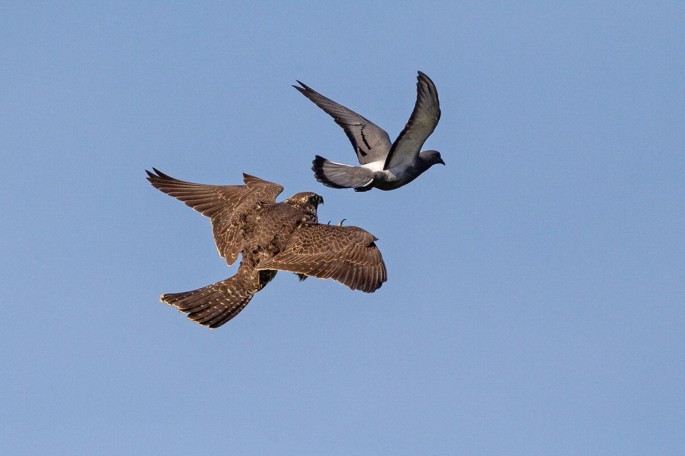In this striking image of two birds in flight against a clear blue sky, the foreground features a dark gray and white pigeon-like bird with darker gray or black wing and tail tips. The bird's wings are up and spread wide, revealing white underneath with a distinctive black line along the wing tips. Its back is white, and its fanned tail transitions from gray to black at the edges.
  
Trailing behind and seemingly in pursuit is a larger bird resembling a hawk, characterized by varying shades of brown. Its wings are fully extended, displaying a combination of lighter and darker brown hues with a pointed beak and vividly detailed horizontal lines on its fanned-out tail feathers. The hawk appears to be on an attack trajectory, its talons reaching forward towards the unaware smaller bird, capturing a moment of raw avian dynamics against a seamless azure backdrop.